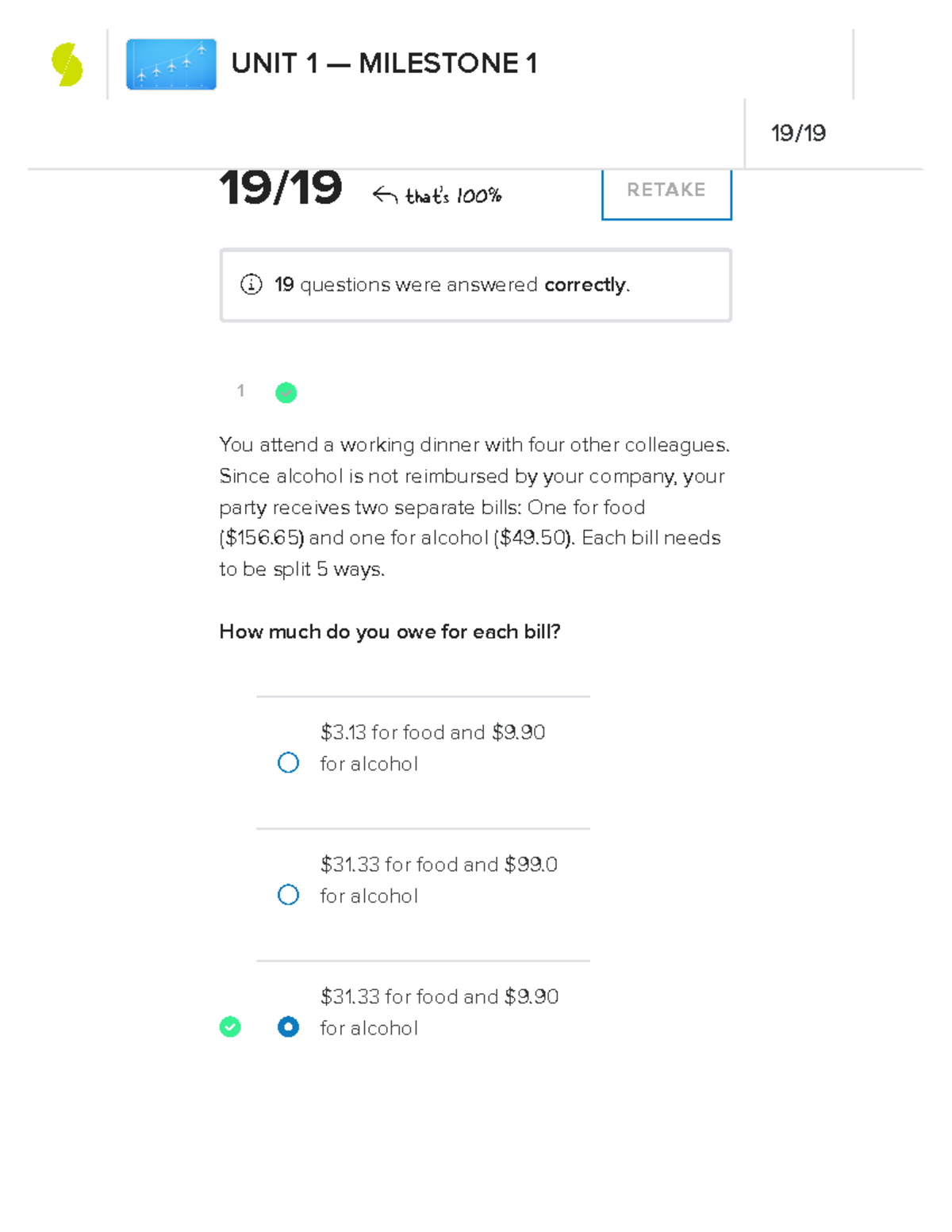This image depicts a screen capture from a cell phone showing progress in an educational application. At the top of the screen, it reads "Unit 1 – Milestone 1," indicating the section of the course. Beneath this heading, the score "19/19" is displayed, signifying perfect accuracy at 100%. Adjacent to the score, there is a white button with a green border, which is labeled "RETAKE" in uppercase gray letters.

Below this button, a text box states, "19 questions were answered correctly." Further down, the screen presents a scenario, suggesting the user is preparing for another test. The scenario describes a working dinner with four colleagues, noting that alcohol expenses are not reimbursed by the company. Thus, the bill is split into two: one for food costing $156.65 and one for alcohol at $49.50, both needing to be divided equally among five people.

The question posed is, "How much do you owe for each bill?" Three options are presented:

1. $3.13 for food and $9.90 for alcohol.
2. $31.33 for food and $9.90 for alcohol. *(this is the correct choice)*
3. Another non-listed option.

The correct and selected answer is highlighted with a bullet: "$31.33 for food and $9.90 for alcohol."

This detailed screen capture illustrates the completion and perfect scoring of a milestone, as well as engaging the user with a math-based scenario to further test their understanding.